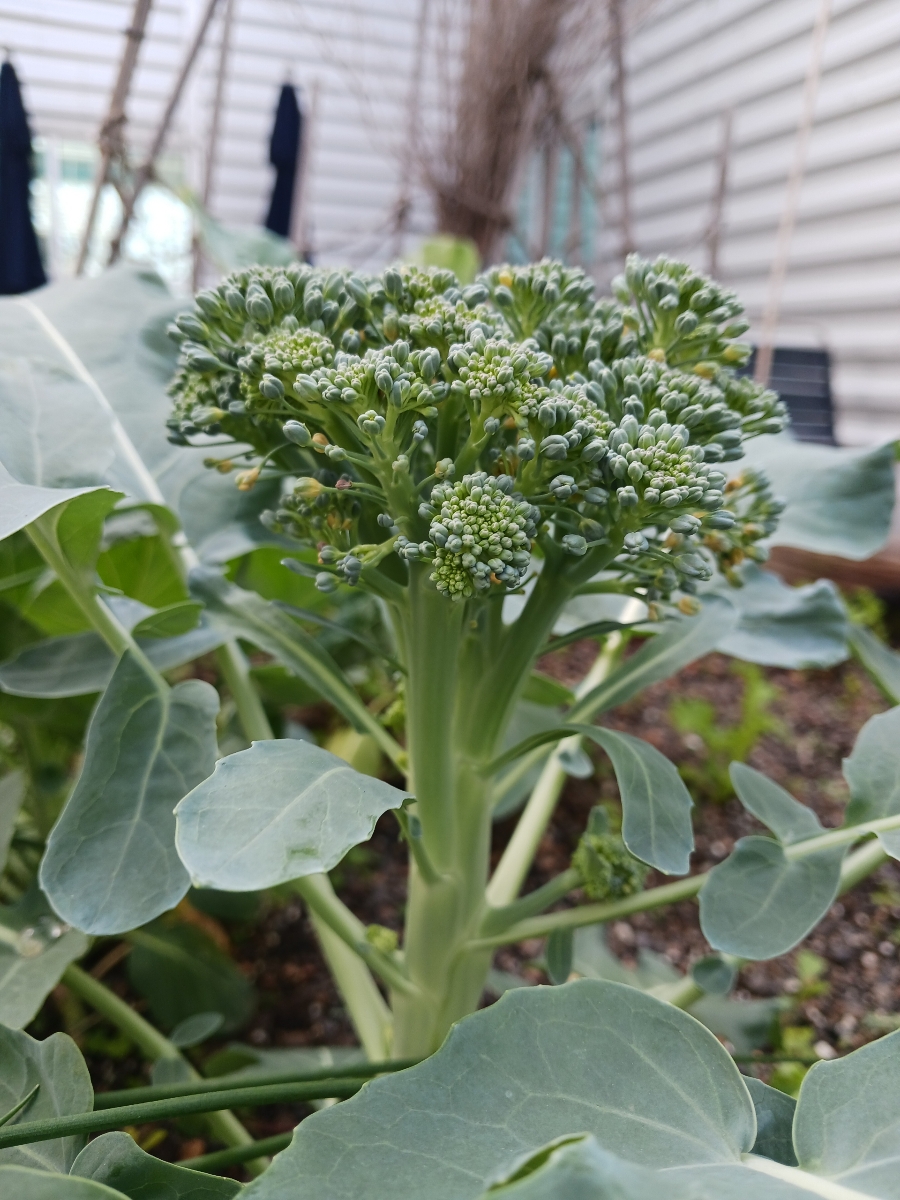This detailed color photograph features a tall, green plant centrally positioned against the backdrop of what appears to be a storage area or greenhouse. The focal plant has a thick stalk and medium-sized leaves, topped with structures resembling small, green broccoli florets, though it may not actually be broccoli. The plant stands out amidst a scattered brown dirt ground, which also contains speckles of tan rock sediment. Surrounding the main plant are numerous dark green leaves from other budding plants. In the background, you can observe brown, feather-like objects that look like decorative pieces, hinting at a garden center or similar setting. The right side of the image is bordered by white blinds, enhancing the enclosed feel of the space. There are no textual elements, people, animals, or motorized objects visible in the photograph, ensuring the viewer's attention remains on the vibrant vegetation.